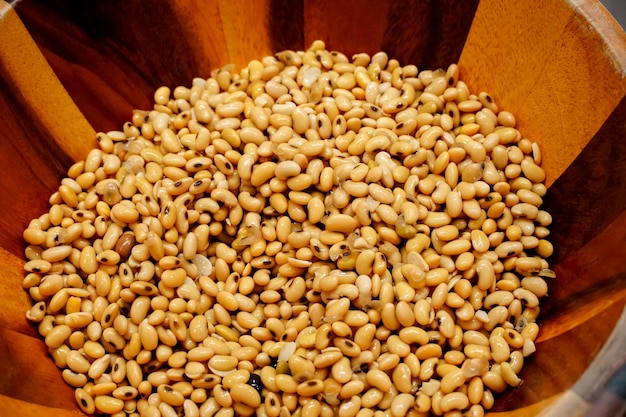This is an aerial photograph of a large, round wooden mixing bowl, showcasing its deep and wide structure. The bowl is crafted from two-toned wood, featuring horizontal stripes that alternate between light and dark brown, creating a striking visual contrast. Inside the bowl, which appears to be about one-third to one-half full, is a generous quantity of black-eyed peas. These beans are uniformly oval-shaped with rounded tops and bottoms, predominantly light beige in color with distinctive black speckles on the underside. The beans have a lustrous sheen, suggesting they have been washed or possibly cooked. The photograph captures the beans intermingled, some showing the black speckle while others do not, highlighting the varied orientation of the beans. Only part of the bowl's edge is visible, emphasizing the centrality of the beans, and the image border is rectangular, guiding the focus to the textured and polished appearance of the beans against the wooden bowl.